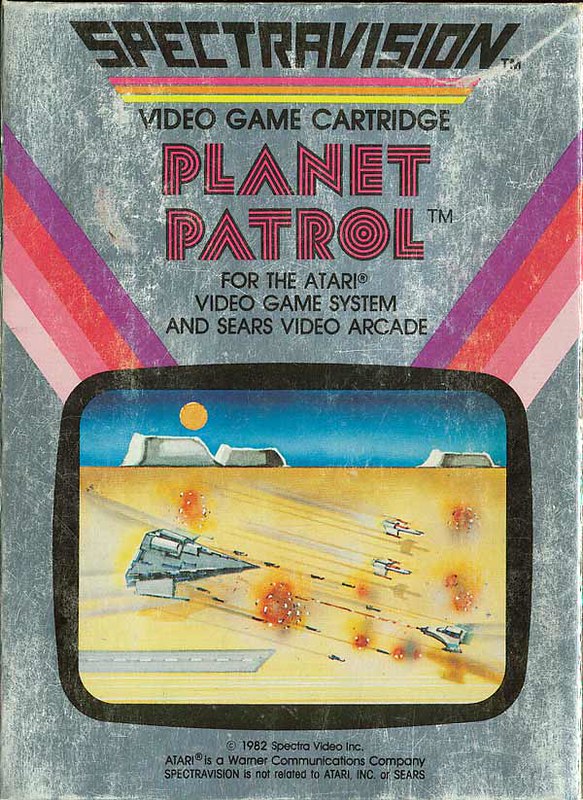The image is a cropped photograph of an aged video game cover, specifically for a game titled "Planet Patrol." The cover itself shows significant signs of wear and tear, featuring a predominantly grey background marred by numerous white marks, indicative of its old, worn condition. Dominating the lower center of the image is a depiction resembling a black screen, upon which a snapshot of the game's retro gameplay is portrayed. In this scene, a spaceship navigates from left to right, firing at enemy spacecraft situated on the right side of the screen. This action unfolds over a desert landscape, beneath a sky adorned with grey mountains and a prominent yellow sun. Adding to the vintage aesthetic, vaporwave-inspired lines radiate from the top left and right corners of the screen representation, enhancing the nostalgic feel of this classic video game cover.